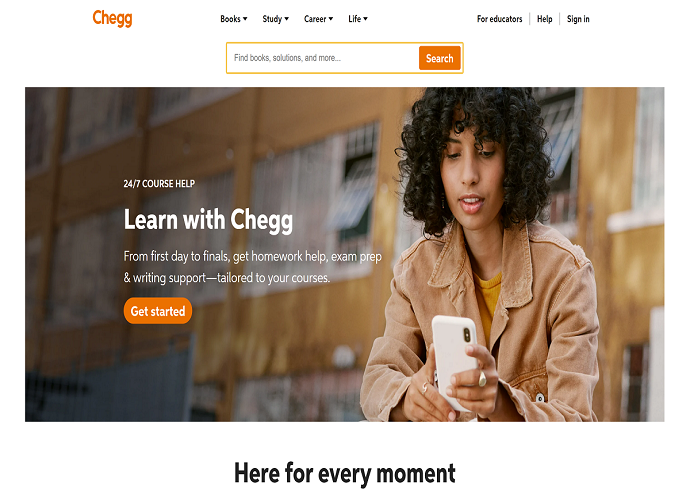This detailed caption describes a promotional image for Chegg displayed on a webpage. 

---

The color image, sourced from a webpage titled "Chegg" written in orange at the top left corner, features various navigational tabs. These tabs—Books, Study, Career, and Life—are displayed in black. On the top right corner, options for Educators, Help, and a Sign-In button are provided. An orange text box below includes a search bar labeled "Find books, solutions, and more" with an accompanying white-text search button.

The image promotes Chegg, highlighting its 24/7 course assistance, including homework help, exam preparation, and writing support tailored to students' needs. An orange clickable button reading "Get Started" appears underneath the promotional text.

The image captures a classroom scene where a young female student, dressed in a brown denim jacket, is engrossed in her white cellular phone, looking down at the screen. At the bottom of the image, the tagline reads, "Here for every moment."

---